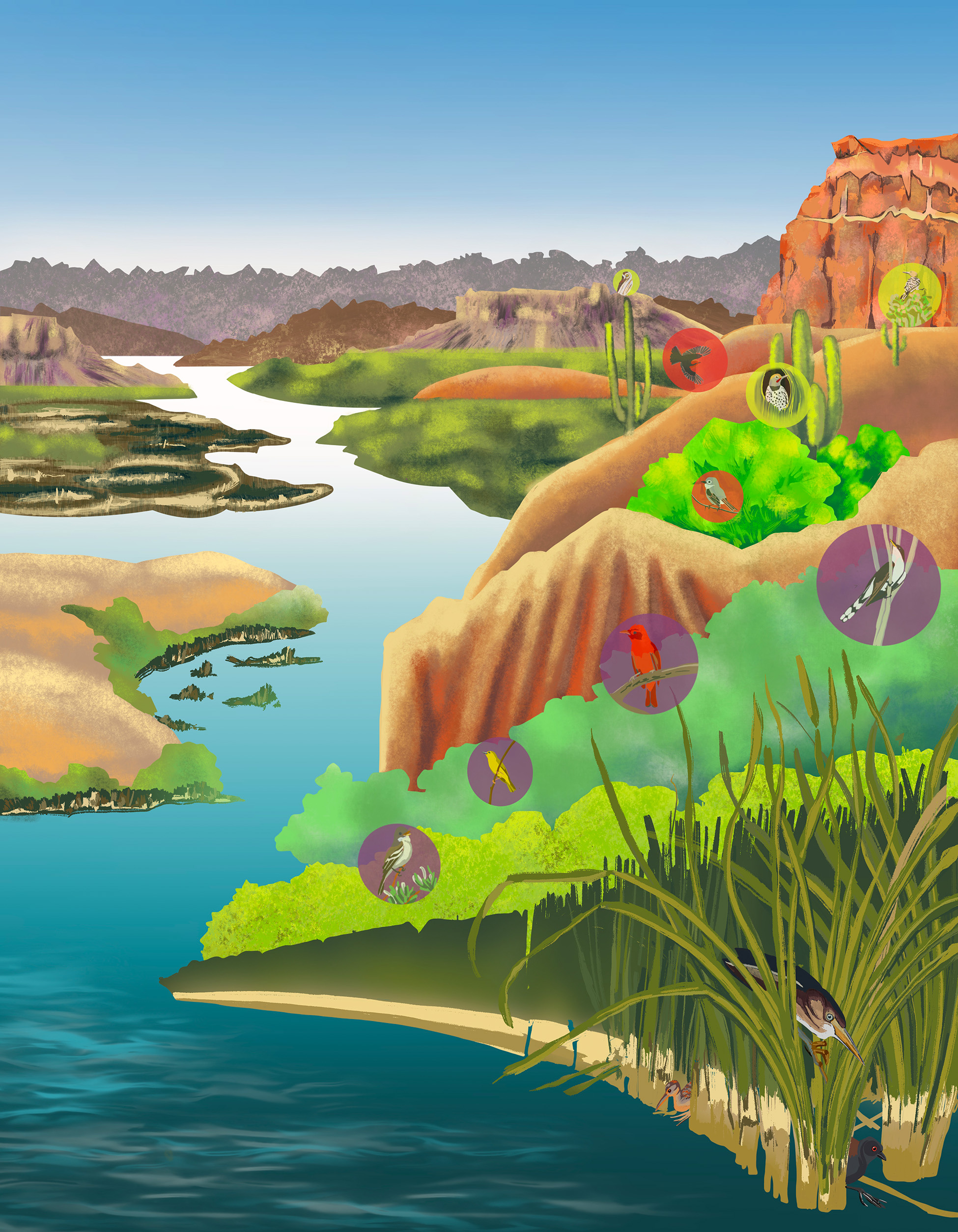The digital illustration portrays a detailed outdoor scene featuring a river winding through an arid mountain range and a swampy area in the foreground. The right side of the river is bordered by rough bushes and water-loving plants. The left side exhibits a sandy landmass transitioning into a darker, more fertile soil. Multicolored circles scattered along the greenery depict various birds, with one circle showing a red bird, another a yellow bird, and a green-circled cactus featuring a white bird. Additionally, a little duck hides among the reeds at the front. The scene also hints at the presence of mosquitoes, crawfish, and other insects typical of this habitat. The river extends about three-fourths up the image, leading to a steep, rounded mountain range in the background.